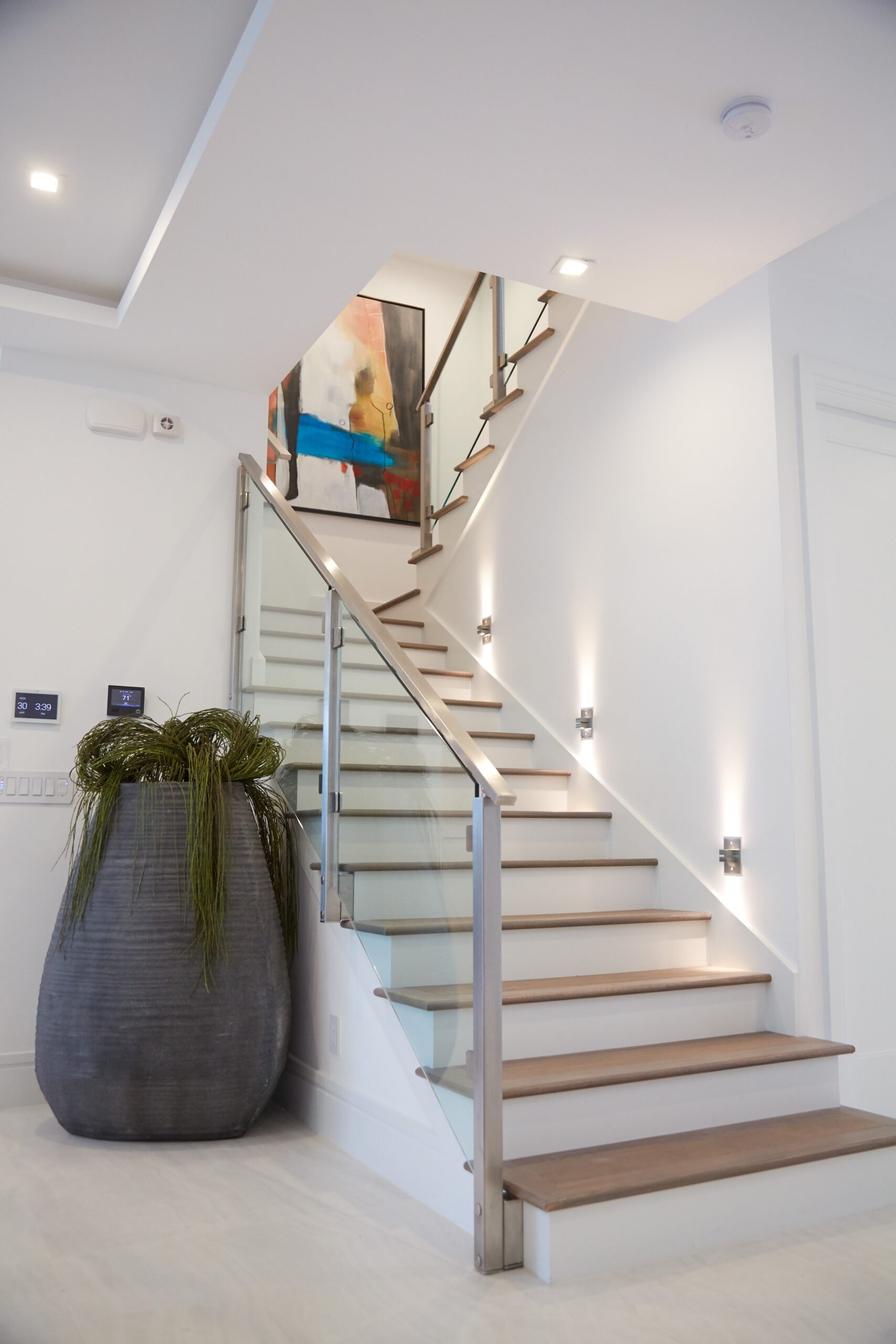This photograph depicts an interior space that could be a modern house or an art studio, characterized by its minimalistic and elegant design with predominantly white and light gray tones. The focal point is a stylish staircase that ascends from the bottom right towards the middle and then turns upward to the top right. The staircase features white risers with light brown wooden steps and is flanked by a sleek glass banister with a metallic silver handrail on the left side.

To the left of the staircase, a tall, gray urn standing about four to five feet high holds cascading greenery, adding a touch of nature to the scene. The gray flooring complements the light gray walls that stretch throughout the space. At the landing of the first flight of stairs, an abstract painting with an array of colors including black, yellow, white, blue, and gray sits in a black frame, providing a striking contrast against the muted backdrop. Recessed lights illuminate the upper part of the image, while smaller night lights line the staircase, hinting at a twilight setting. The overall atmosphere is both contemporary and serene, seamlessly blending art and function.